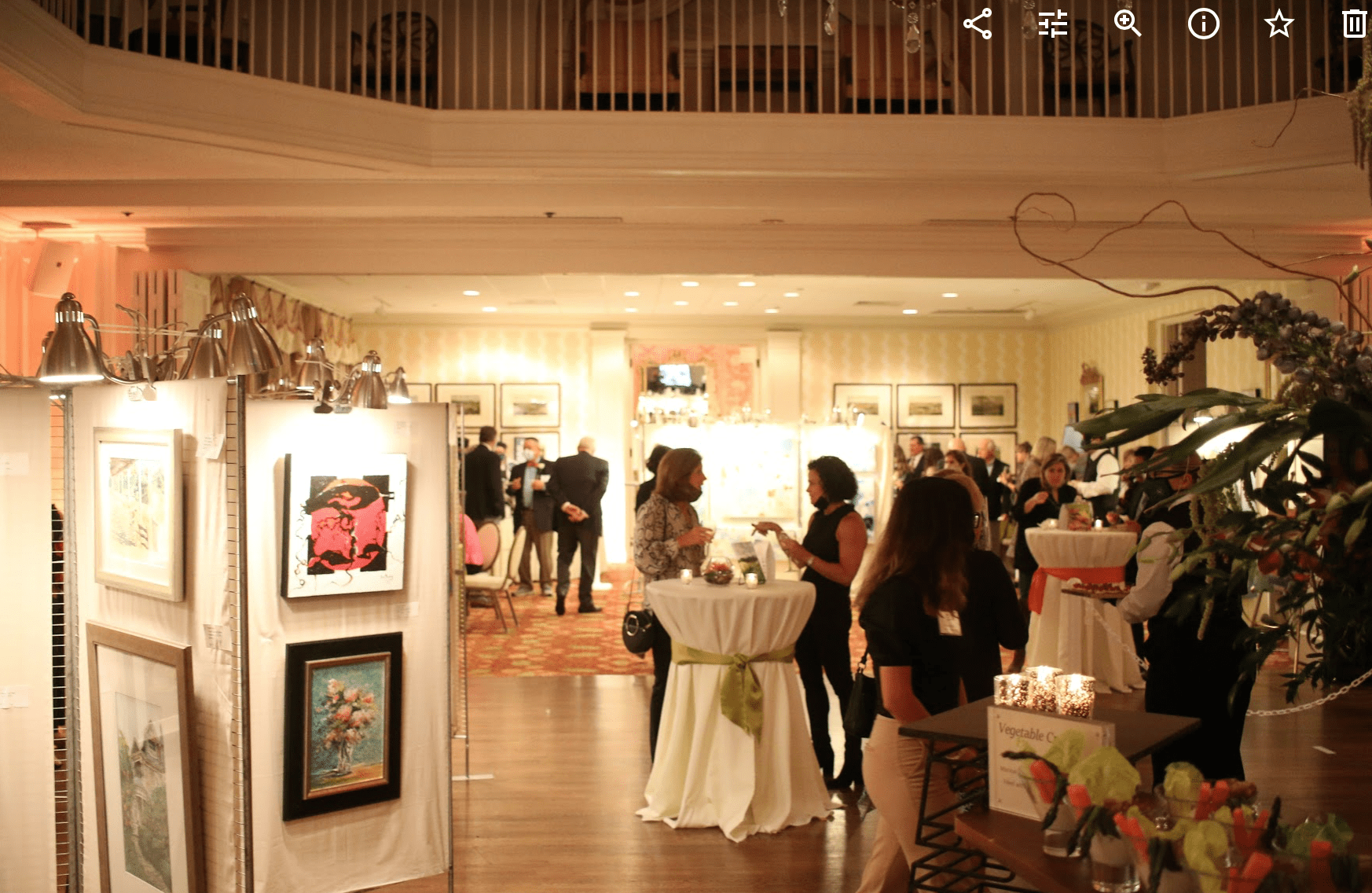A rectangular image, likely captured on a phone or viewed on a computer, features various symbols in the upper right corner, forming a nearly triangular shape. These symbols include two connected lines, horizontal lines, and icons such as a search icon, an eye in a circle, a star, and a trash can symbol.

The scene depicted shows a lively art gallery or exhibition. The gallery's ceiling is adorned with numerous lights focused on a variety of art pieces, creating a well-lit and inviting atmosphere. Guests are seen mingling and engaging in animated discussions around cocktail tables, adding a sense of community and interaction to the event. The tables are adorned with candles, casting a warm and intimate glow. Additionally, there is a dedicated drinks table, also decorated with candles, enhancing the ambiance and providing refreshments for the attendees.